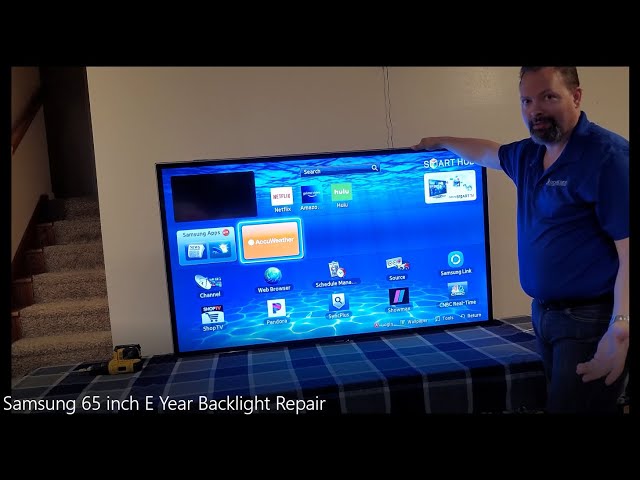The image appears to be a screenshot from a video tutorial featuring a large 65-inch Samsung TV monitor positioned centrally on a table covered with a blue and white checkered tablecloth. At the bottom of the image, there is a caption reading "Samsung 65-inch E-Year Backlight Repair." The monitor, displaying what seems to be a computer home screen filled with various small, unreadable icons, is placed against a plain white wall. To the left side of the wall, a set of stairs extends into the darkness. A power drill is lying on its side next to the monitor. On the right side of the image, a middle-aged Caucasian technician with a short beard and mustache, dressed in a blue polo shirt and jeans, stands next to the TV. His left arm is at his side while his right arm is reaching out to hold the top corner of the screen. The technician is looking directly at the camera, suggesting he is engaged in explaining a repair procedure.